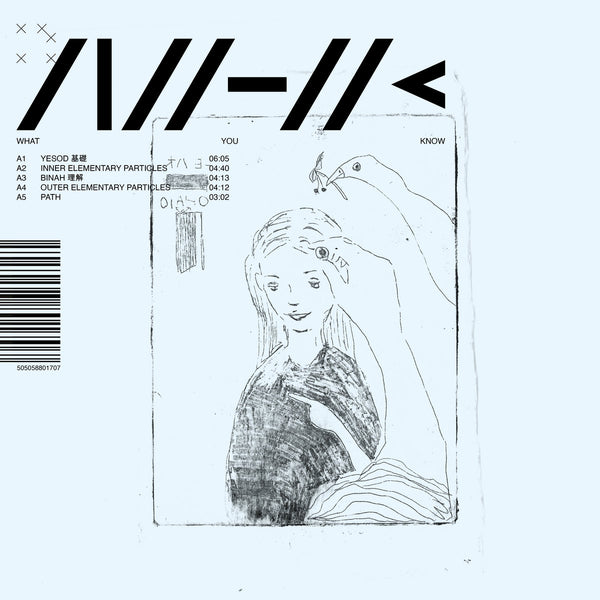The image appears to be a detailed cover, potentially for a magazine, CD, or comic book, featuring a central rectangular pencil sketch illustration against a pale blue background. The sketch depicts a young woman, dressed in a dark top, looking down with a slight yet gentle expression. Another individual is seen placing a small flower in her hair while pointing at something with a finger. Above her, there's a white bird, resembling a swan or a goose, gracefully holding another flower in its beak.

To the top and left of the frame, the image incorporates various elements including text and symbols. The upper right corner features the words "you" and "no," alongside certain numbers. The upper left corner is marked with black stripes and X-shaped markings, which add a unique graphical element to the composition. Along the left side, there is a list of text with hierarchically arranged elements: "A1, A2, A3, A4, A5," and phrases such as "yes, LD, inner elementary particles," and "now outer elementary particles and path." These might suggest song titles and run times or segmented chapters, contributing to the structured narrative of the piece.

The cover also includes Asian characters, possibly reinforcing the notion of Japanese animation influences, and a barcode structure situated on the left side, hinting at its commercial nature. The top of the image is adorned with slashes and dash characters, further emphasizing a sophisticated design language.

Overall, the detailed composition amalgamates the delicate pencil sketch of a girl with layered textual and graphical elements, presenting a fusion of aesthetic and possibly thematic storytelling.